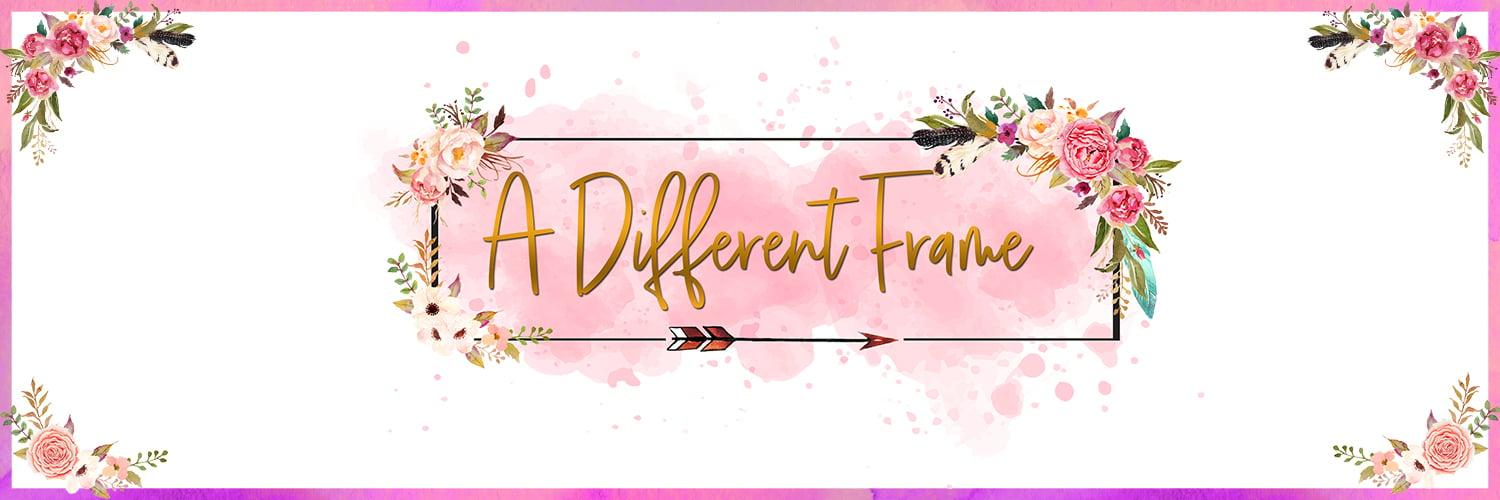The image is a digitally designed advertisement banner presented as a long horizontal rectangle with a 4:1 aspect ratio. The banner features a thin, gradient border that transitions from pink to lilac. Each corner of the rectangle showcases a bouquet of flowers, prominently roses with green leaves, rendered in varying shades of pink and dark pink. In the center of the banner sits a smaller black rectangle outlined in thin black ink. Inside this smaller rectangle, cursive gold text reads "A Different Frame," standing out against a backdrop of a pink ink blotch. This central black rectangle is accompanied by floral bouquets in the upper left, upper right, and bottom left corners. Additionally, beneath the central text, there is a decorative arrow pointing to the right, designed with an arrowhead on one end and dual sets of quivers on the other. The overall effect is an elegant and cohesive design primarily featuring gold, pink, and floral elements.